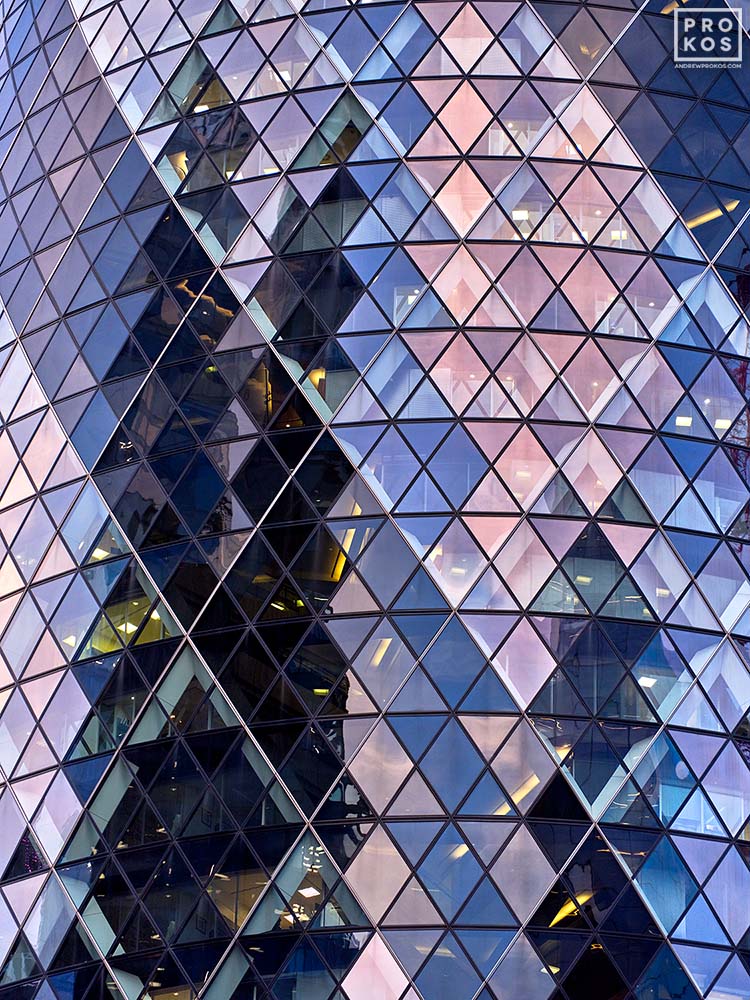This detailed close-up photo captures a stunning skyscraper adorned with numerous glass panels shaped like triangles and diamonds. The windows exhibit a captivating range of colors, including hues of pink, blue, light pink, light blue, dark blue, and dark pink, with some panels being transparent, allowing glimpses inside revealing illuminated office spaces. Metal poles crisscross behind the glass, adding to the intricate design. The building reflects elements of its surroundings, enhancing its unique aesthetic. The name "ProCost" is prominently displayed at the top right, possibly indicating the company associated with the building.